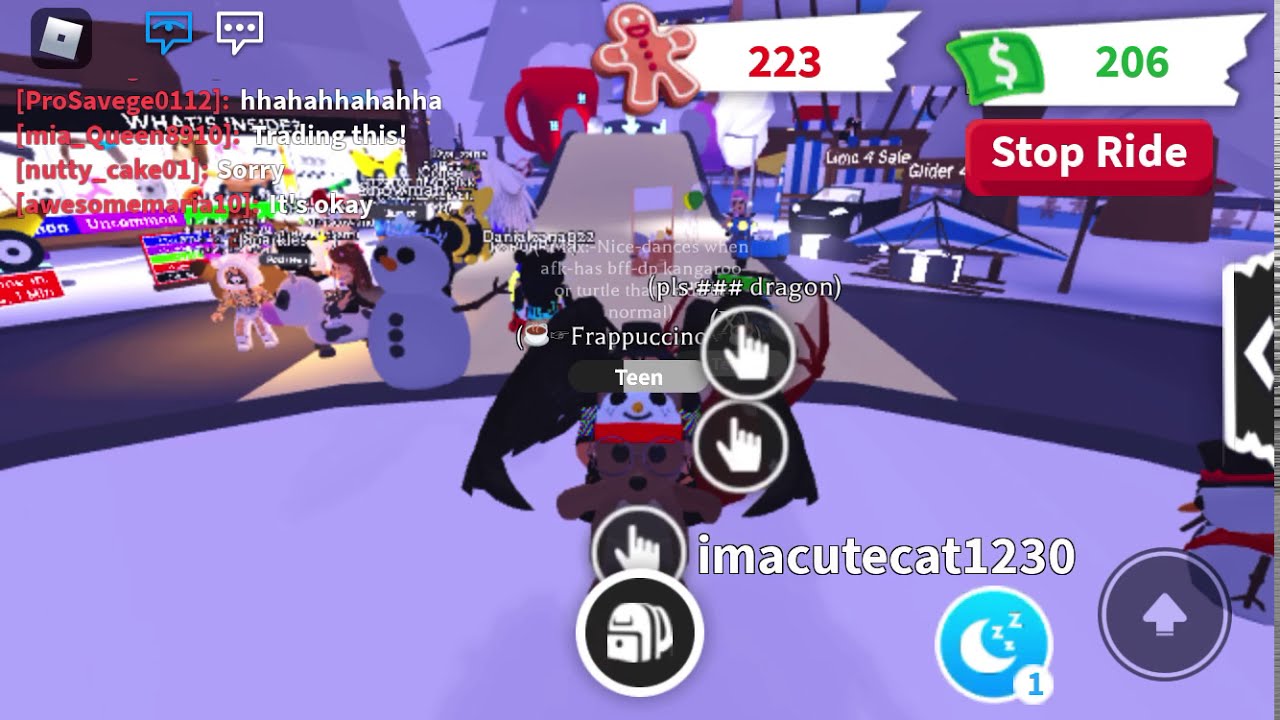In the image, there's a vibrant screen capture of a social virtual reality (VR) video game, likely designed for Oculus or similar VR platforms. The scene is set in a lively environment that blends elements of a nightclub and an outdoor ski resort. The floor has a distinct purple hue, contributing to the ambient lighting that envelops various themed avatars. Players are represented as diverse characters, such as a snowman, a seal, a gingerbread man, and even a cheetah-like figure wearing a furry hoodie, all interacting with each other.

Above each avatar, snippets of dialogue float, showcasing an engaging chat system. Usernames appear in red followed by white text, expressing jovial and conversational exchanges. For example, ProSavage0112 laughs with "ha ha ha ha," while Mia Queen mentions "trading this," and Nutty Cake and Awesome Maria 101 exchange apologies with "sorry" and "it's okay," respectively.

The upper left corner features a dedicated chat area displaying these ongoing dialogues. A gingerbread icon with '223' on the top left and an adjacent text box with an eye symbol can be seen. Additionally, there's a 'Stop Ride' button on the right side, indicating interactive elements within the game. A notable white slide in the background further adds to the festive, winter, and possibly holiday-themed aesthetic of the environment.